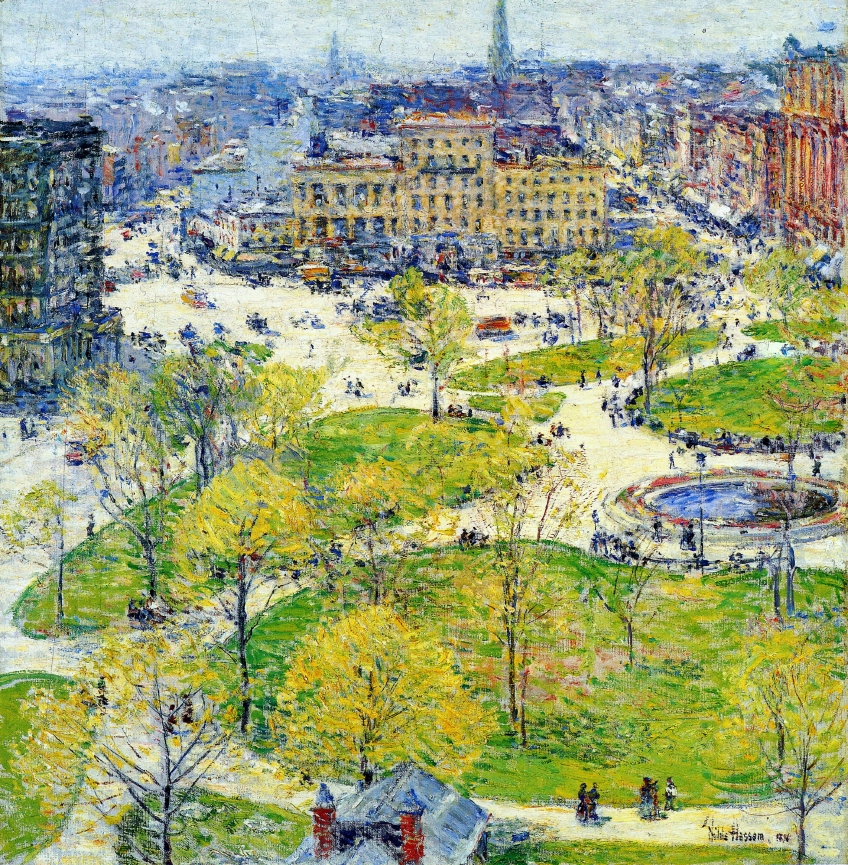This impressionistic oil painting depicts a bustling city park on the outskirts of a town during the day. Dominating the foreground, the park is adorned with lush green trees, bushes, and expansive grassy areas. Central to the scene is a round fountain, surrounded by scattered groups of people leisurely strolling. At the bottom middle of the composition, a building with distinctive gray gabled roofs and two red chimneys sits prominently on a verdant plot, framing the human activity.

The background is a cityscape marked by diverse architectural elements. A tall yellow building commands attention at the center, flanked by a darker multi-story apartment building on the left and a series of houses along a receding street on the right. Behind these structures, a tower emerges against the gray sky, anchoring the horizon. Notably, a horse and buggy add a touch of movement near one of the buildings, enhancing the scene’s dynamic quality. The artist's signature, seemingly "THASSAM," is elegantly tucked into the bottom right corner of the painting, next to more painted people, solidifying the artwork's authenticity and the artist's presence.